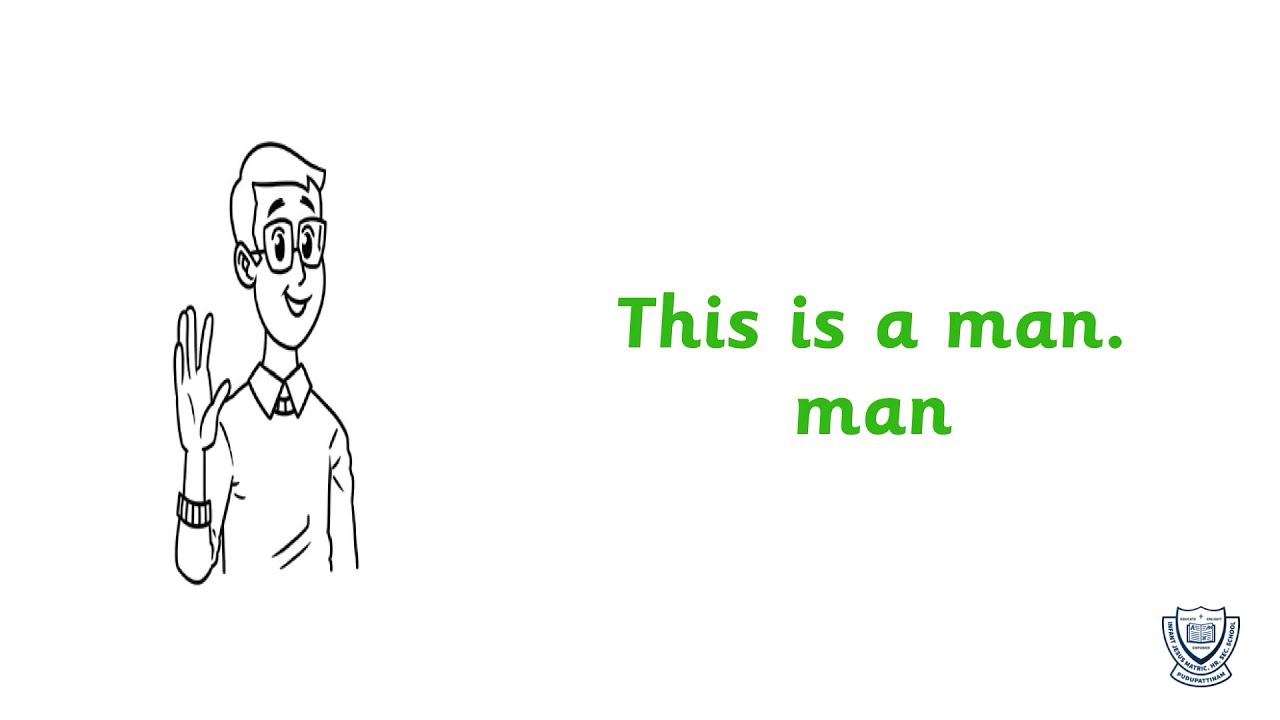This image features a simple, clean design with an all-white background. On the left side, there is a black-and-white cartoon drawing of a man from the waist up. He has short hair with black outlines and glasses. He's smiling and has large eyes and dark eyebrows. The man is wearing a collared shirt underneath a sweater with long sleeves, and his right hand is raised in a waving gesture. 

In the center of the image, there is green text in two lines: the first line reads "This is a man." and the second line simply says "man." Both lines are center-justified. 

In the lower right corner, there is a black-and-white logo that resembles a shield with a semi-oval base, although its details are unclear and its purpose is not specified.